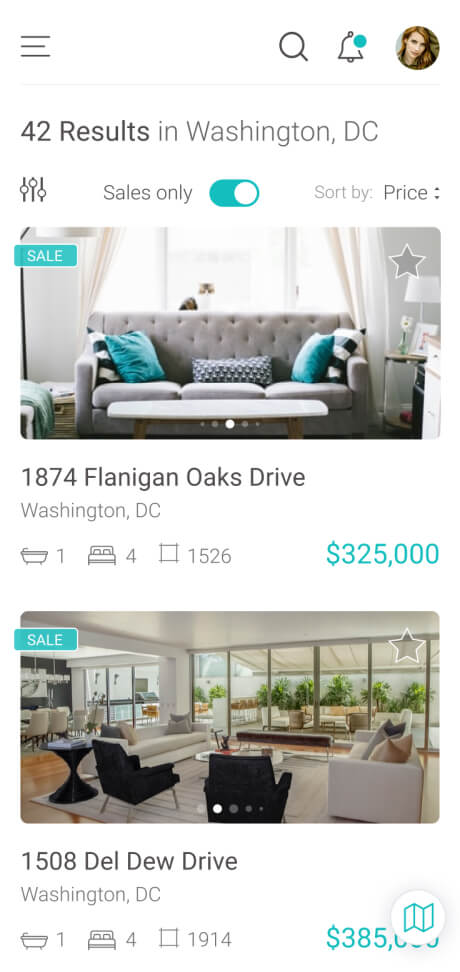This detailed poster displays a variety of home listings in Washington D.C. At the top, it prominently features the title "42 Results in Washington D.C." A blue indicator shows that the "Sales Only" filter is applied. Adjacent to it, on the left, is an additional filter option, while to the right, there is a "Sort by Price" feature.

One highlighted listing is for a property at 1874 Flanagan Oaks Drive. This home, located in Washington D.C., includes images showcasing its bathroom, bedrooms, and overall square footage. It is described as having one bathroom and four bedrooms, totaling 1,526 square feet, with an asking price of $325,000. The listing features an interactive button that allows users to 'star' or 'favorite' this property.

Another featured listing is at 1508 Del Dew Drive. The accompanying image reveals a spacious, inviting living area with two sofas facing each other and a coffee table at the center. To the left, there's an open concept kitchen, and through the glass-paneled area that appears to be an atrium, there is an additional set suggesting an outdoor space. This property includes one bedroom and four bathrooms, stretching over 1,914 square feet, listed at $385,000. 

Additionally, the poster provides a clickable map that directs users to the locations of both properties. At the top-right corner, it indicates that the user is logged in, with a notification alert represented by a blue dot, and a search function is also available for further exploration.